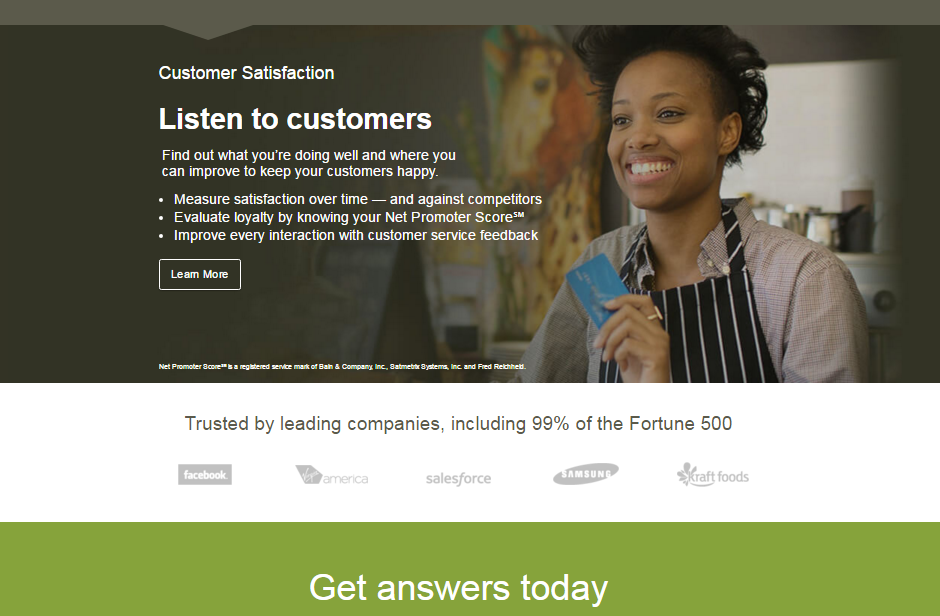A promotional screenshot for a customer satisfaction service, prominently featuring an advertisement aimed at businesses seeking to enhance their customer relations. The ad is headlined with "Customer Satisfaction" and further explains the importance of listening to customers, identifying strengths, and pinpointing areas for improvement to ensure customer happiness. A key visual element includes an image of an African-American woman holding a card, possibly indicating a recent purchase.

The ad highlights that the service is trusted by an impressive array of leading companies, including 99% of the Fortune 500, with notable users such as Facebook, Feed America, Salesforce, Samsung, and Kraft Foods. The advertisement underscores the service's capabilities to measure satisfaction over time and in comparison with competitors, aiming to improve every customer service interaction through valuable feedback.

A call-to-action button, labeled "Get Answers Today," suggests that clicking it would provide further information about the company's offerings and how their services can help businesses effectively gauge and enhance customer satisfaction.